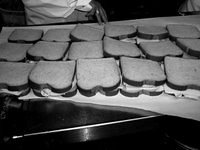A small, black and white photograph captures a meticulous arrangement of 17 sandwiches placed on a large sheet of parchment paper on a black tabletop. The sandwiches are organized into three rows, with five in the first row and six in the subsequent rows. The bread appears to be standard loaf bread, potentially white or wheat, given the varying shades of gray. Each sandwich features some type of lunch meat, possibly ham or turkey, visible through the sandwich layers. The image suggests a preparation area, possibly in a restaurant setting. In the background, a person partially appears, identifiable by a right hand adorned with a ring and dressed in a white shirt or apron, hinting at a chef or food preparer.